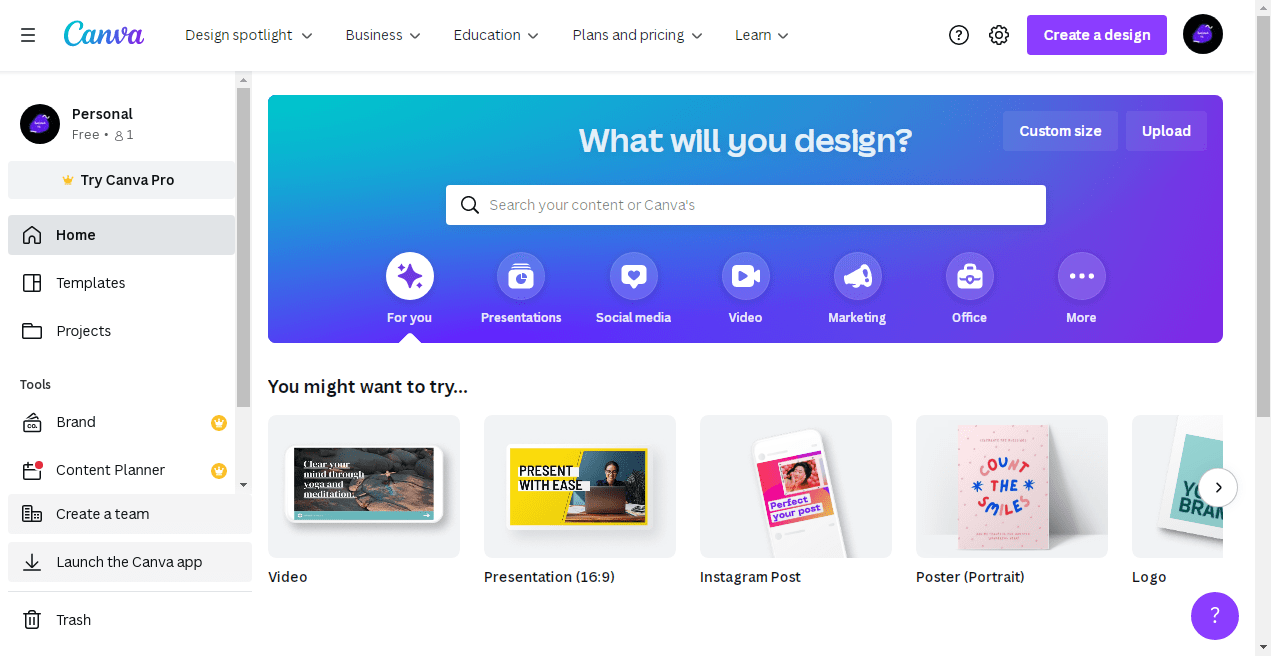A screenshot of the Canva homepage on a personal free account. The webpage prominently displays the header text, "What will you design?" below which lies an array of editable template options. These include categories such as video, presentation, Instagram post, poster, and portrait, designed to inspire creativity. The interface encourages users to explore various design possibilities by offering a versatile platform for creating a wide range of media content.